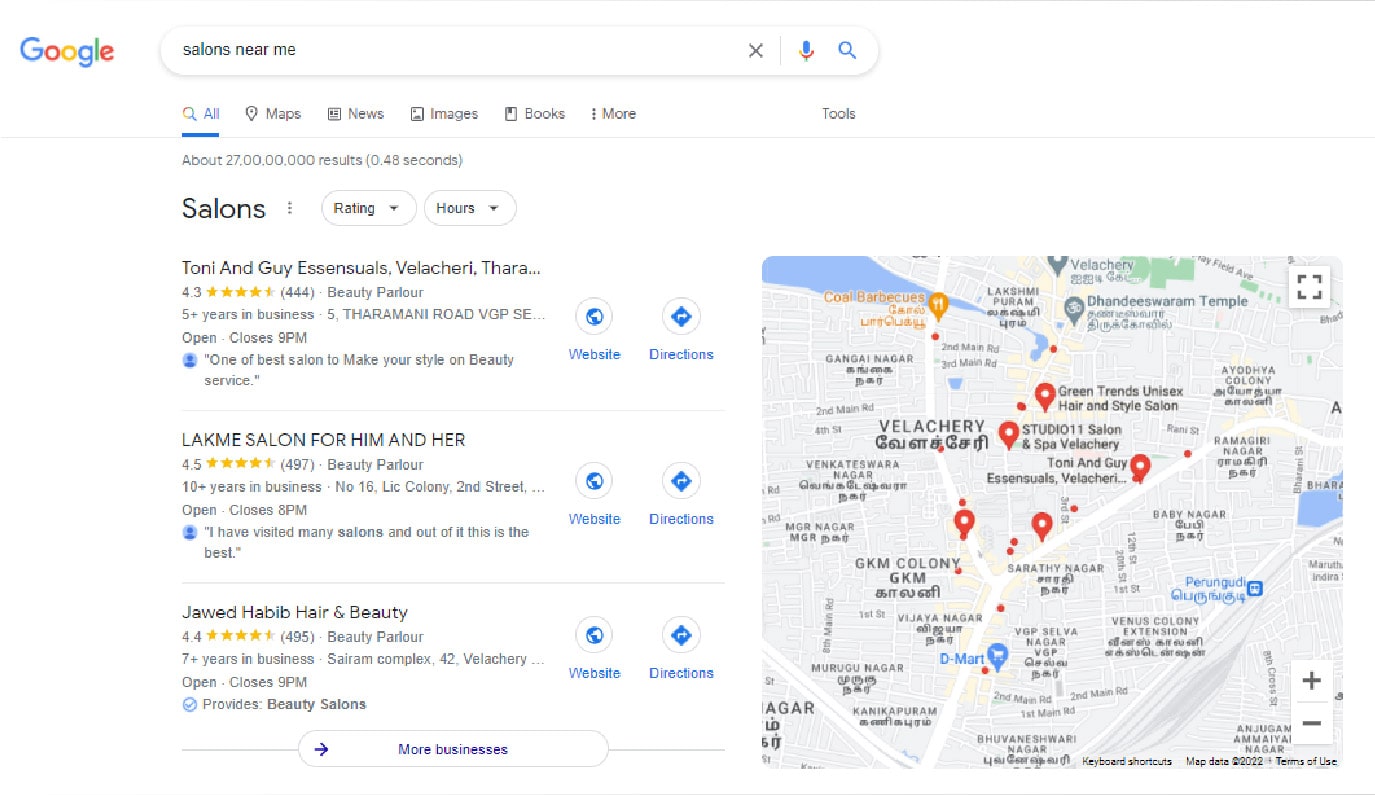This screenshot captures a Google search results page for "salons near me." In the top left corner, the colorful Google logo is visible, followed by the search bar containing the query "salons near me." Below the search bar, there is a row of icons labeled: All, Maps, News, Images, Books, More, and Tools.

Beneath these icons, a heading reads "Salons" in bold black text, followed by "writing in hours." The page lists several salon options, starting with "Tony and Guy Essentials," followed by "Lakmé Salon for Him and Her," and "Jawed Habib Hair and Beauty." Each listing features circular icons next to it for accessing the salon's website and obtaining directions.

On the right side of the screen, a map displays the locations of the listed salons, marked with red pins. The map shows a total of six points: five red pins representing salons and one blue dot indicating a supermarket. Additionally, an orange marker denotes a restaurant situated near a lake in the upper left-hand corner of the map. Streets and other named locations are also visible, providing a comprehensive overview of the area.